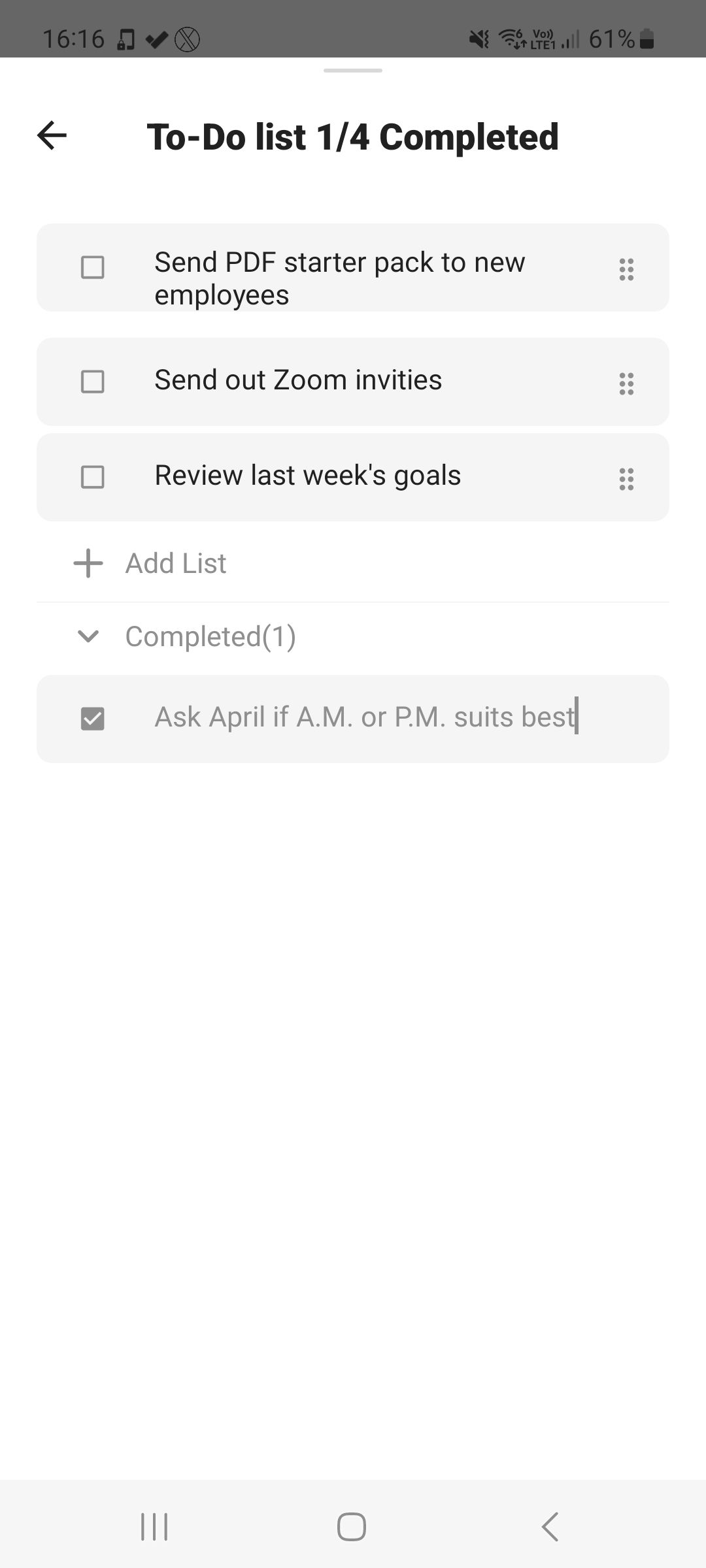The image depicts a to-do list on a smartphone screen. At the very top, the number "1616" is blacked out. A small music note icon, a check mark, and an X inside a circle are visible alongside an X-ed out sound bar, indicating muted sound. Wi-Fi bars are present, along with a battery percentage of 61%.

The bottom section of the screen shows the to-do list interface. Only one out of four tasks is completed, as shown by "1/4 completed" at the bottom. An arrow pointing to the left is also visible. The tasks listed, each accompanied by an empty checkbox, include:
1. "Send PDF starter pack to new employees."
2. "Send out Zoom invites."
3. "Review last week's goals."

The list is displayed within a gray-shaded area atop a white background. Nearby, a plus sign allows for the addition of new tasks. A down arrow button labeled "completed" with the number "1" in parentheses is also visible. Furthermore, there is a grayed-out box with a white check mark containing the text "check off," followed by a task that reads, "Ask April if AM or PM suits best."